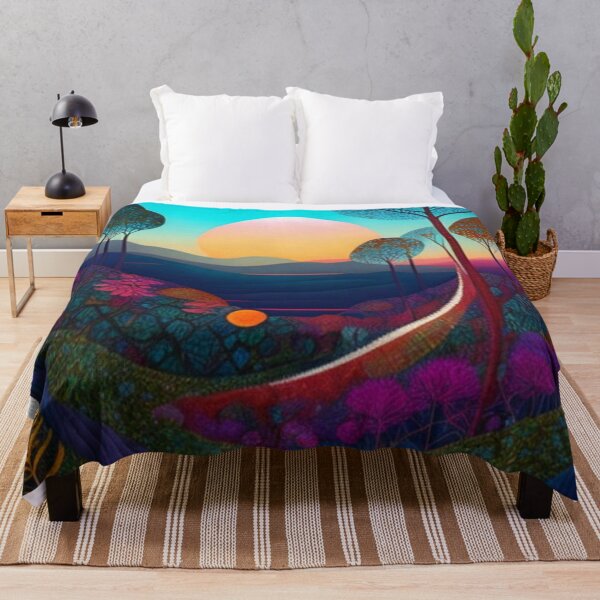This is a perfectly square image of a bedroom, which could be either a painting or a photograph. The room’s background wall is gray and features a white footboard. The floor is a very light wood. Dominating the center of the image is a double bed adorned with white pillows and a multicolored comforter. This comforter depicts an intricate outdoor scene with a blue sky, a large setting sun, trees with brown trunks and blue leaves, and a mix of light greens, reds, oranges, and purples. The bed rests on a brown and white striped rug. To the right of the bed, a tall green cactus grows from a wicker basket with handles. To the left, there is a wooden nightstand with a brown top and a drawer, supporting a black lamp. The foot of the comforter transitions from a mix of purple flowers and green foliage to blue sections with shapes like triangles or ovals, possibly representing rocks or water. The midsection shows umbrellas akin to those found on a beach, and the upper section has gray mountains or hills, culminating in a mostly blue sky with a prominent yellow sun.